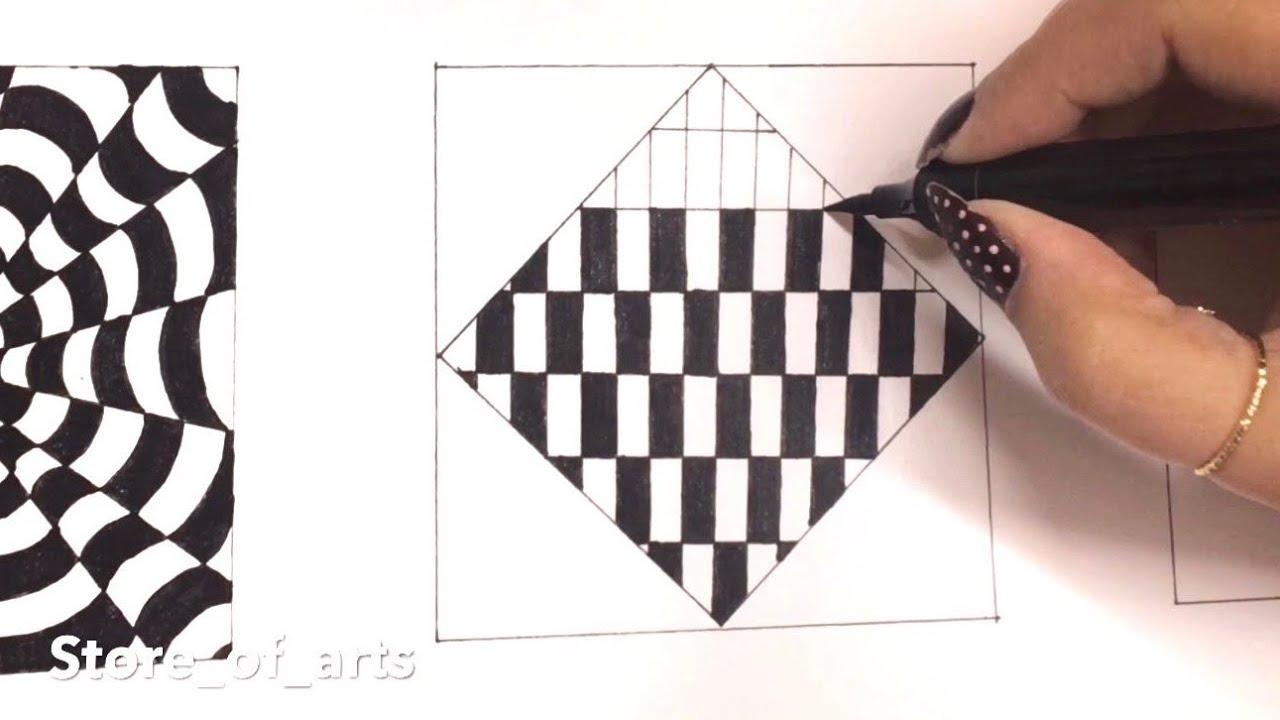The image is a detailed drawing featuring a close-up of a woman's hand, identifiable by her long fingernails painted dark with white dots. She wears a gold ring on her thumb and is holding a black pen. In the center, she is meticulously coloring in a black-and-white square that contains a diamond-shaped pattern. This diamond is filled with rows of rectangles, which she is coloring alternately black and white, creating a checkerboard effect. The top two rows of the diamond remain uncolored. On the left side of the drawing, there is a finished, intricate, spiral-like design with wavy, black-and-white alternating patterns. Below this on the left, in white font, is the text "Store_of_Arts," partially obscured by the white background. On the right, partially covered by her hand, is another square, similar in size to others but still unfinished. The overall scene conveys the process of creating detailed, alternating black-and-white patterns.